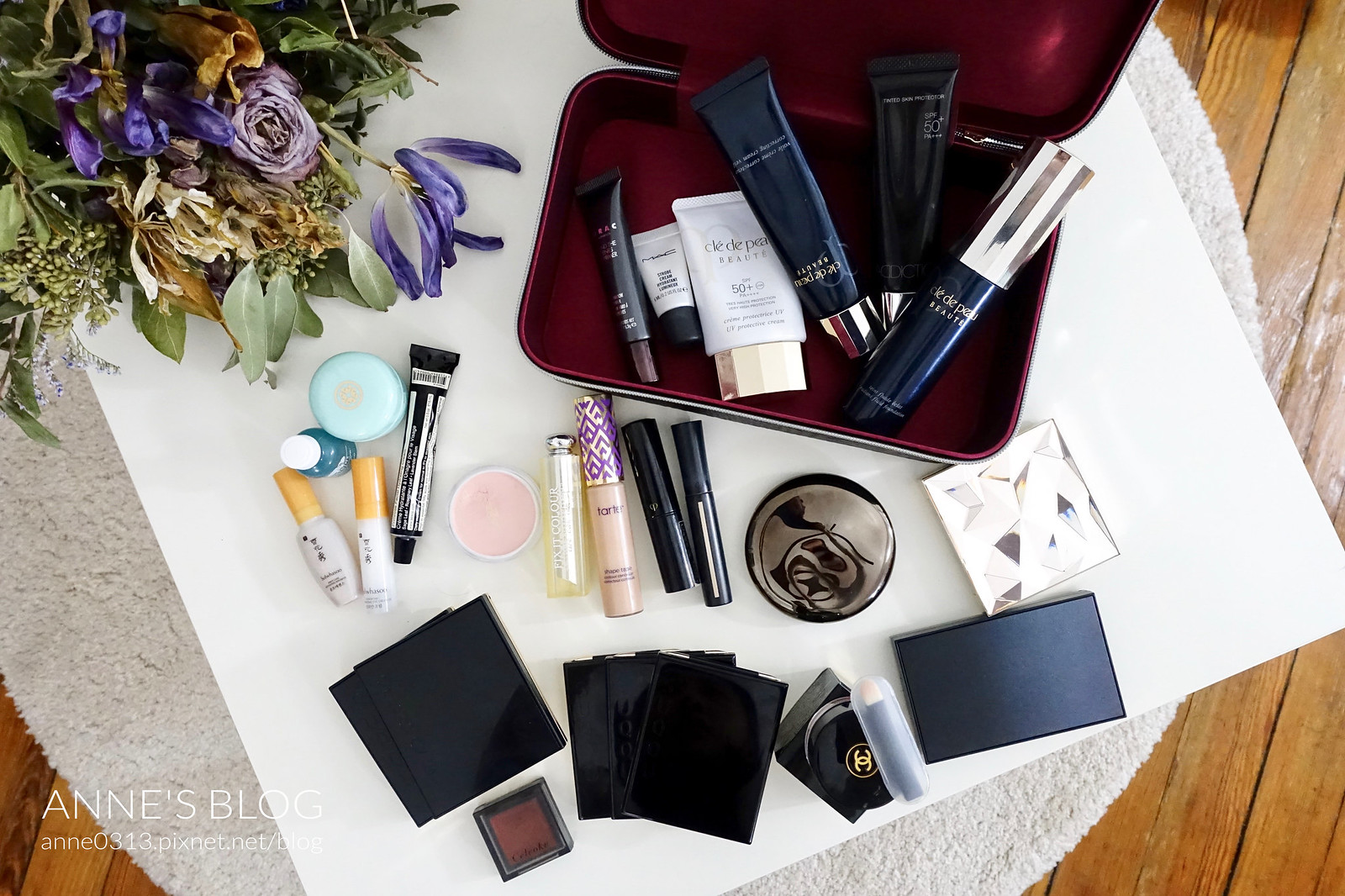The photograph was taken in an indoor setting and depicts a well-organized scene. A light gray round rug is placed on top of light brown hardwood flooring. Centered on the rug is a large, square-shaped white poster board. Arranged meticulously on the poster board are several objects, including makeup products such as lipstick and eyeliner, as well as a couple of small notepads. Additionally, there is a burgundy-colored container case that holds creams. 

The interior of the case is a rich burgundy hue, adding a touch of elegance to the composition. In the upper left-hand corner of the image, a cluster of vibrant purple flowers and lush green leaves adds a natural element. On the lower left-hand corner of the poster board, the text "Ann's Blog" is prominently displayed in white. Just below this text is the website URL "ann0313.pixnet.net.blog," providing a clear reference to the blog. The entire image is presented in a rectangular format, capturing the detailed arrangement perfectly.